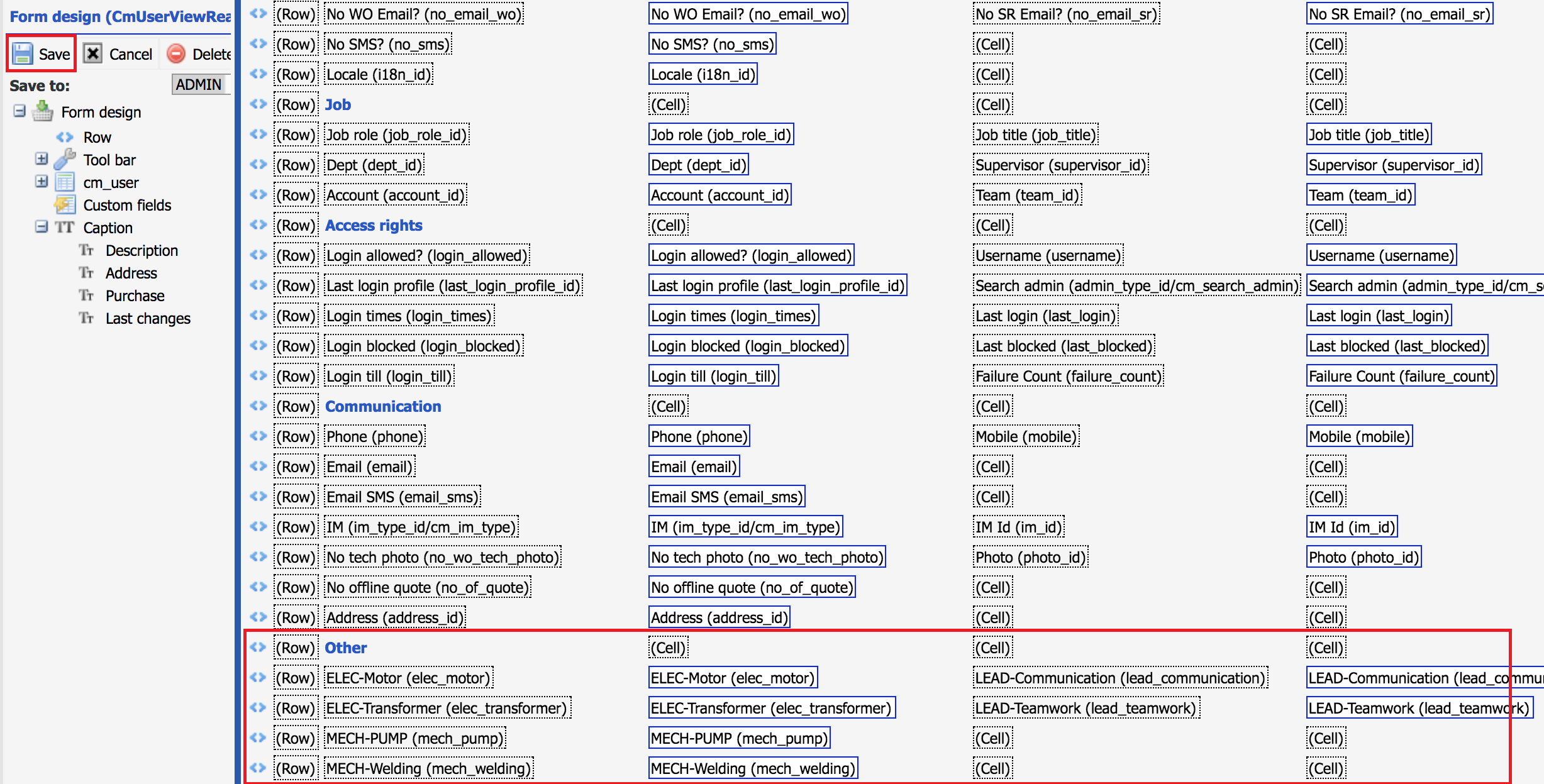The image depicts an online application page. On the left side of the page, there is a vertical frame with the heading "Form Design" written in blue at the top. Below this heading, a "Save" button is highlighted in a red triangle outline. To the right of the "Save" button, there are two more buttons: a "Cancel" button to its immediate right, followed by a "Delete" button.

The main body of the image is set against a pale beige background and comprises 26 rows, each containing four form design elements arranged side by side. Notably, the bottom five rows are encompassed by a red rectangular outline, drawing attention to this specific section.